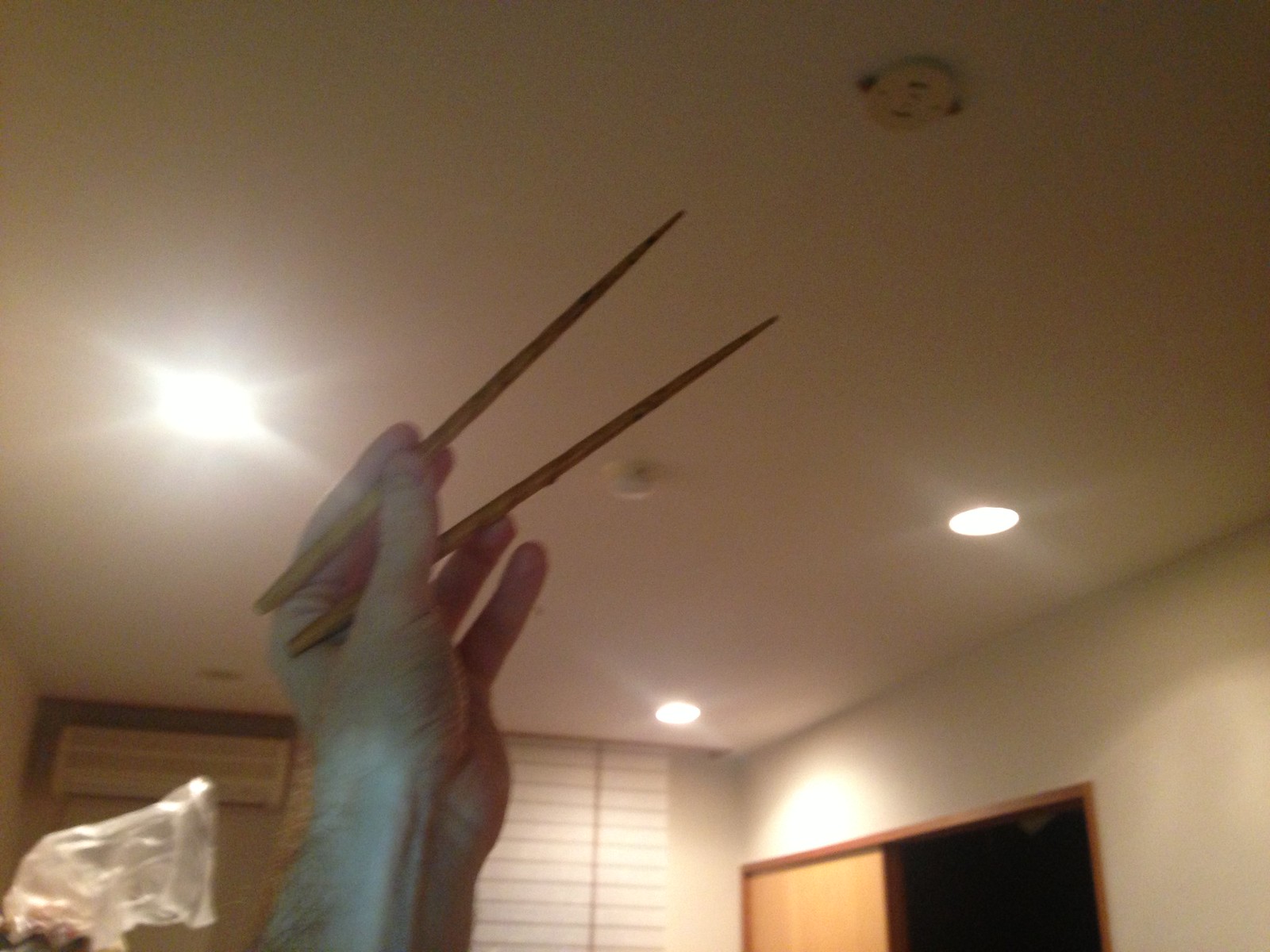The grainy photograph features a male Caucasian hand, characterized by thick brown hair, raising a pair of wooden chopsticks toward a smooth white ceiling with recessed lights, one of which appears to be burned out. The scene suggests an older image due to the low picture quality. In the backdrop, the indistinct surroundings hint at a bedroom, featuring white blinds on a window to the left, a brown sliding closet door to the right, and a faint presence of a plastic bag behind the hand, adding to the ambiguity of the setting.